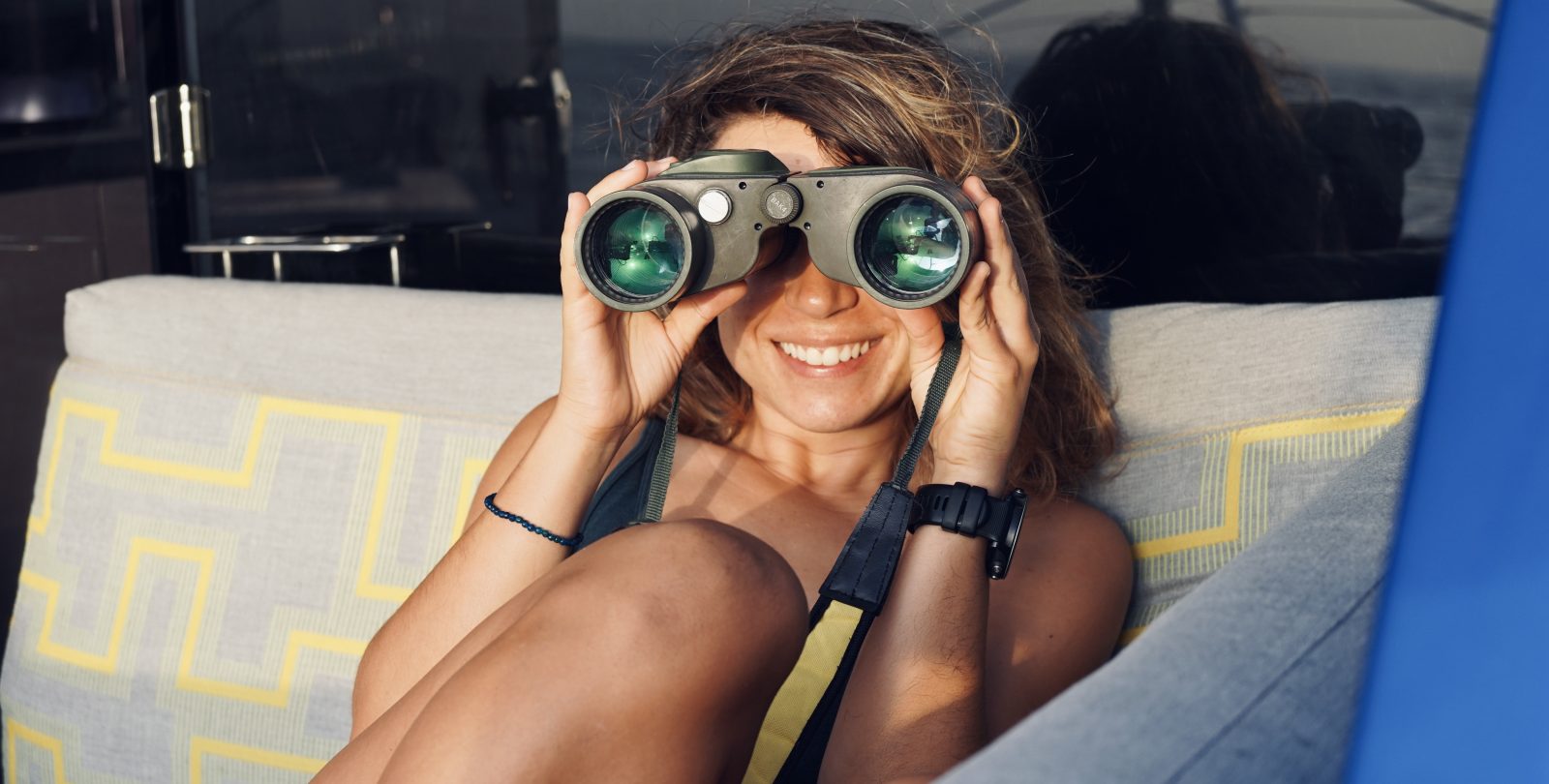In this detailed photograph, a young woman with long blonde hair streaked with lighter shades is seen sitting in a gray chair adorned with white lines on the back seat. She is wearing a black tank top and looking directly towards the camera through a pair of black plastic binoculars, which feature a black leather strap hanging from them and are connected at the center by a bolt. The woman's tanned skin suggests a summery atmosphere, emphasized by her casual attire. On her wrists, she sports a black watch and a thin black bracelet. A small blue curtain can be seen on the right side of the image, adding a touch of background detail. The reflective glass wall behind her captures the back of her head, hinting at the setting's potential indoor-outdoor ambiguity. She smiles slightly, creating a light-hearted and intriguing visual narrative.